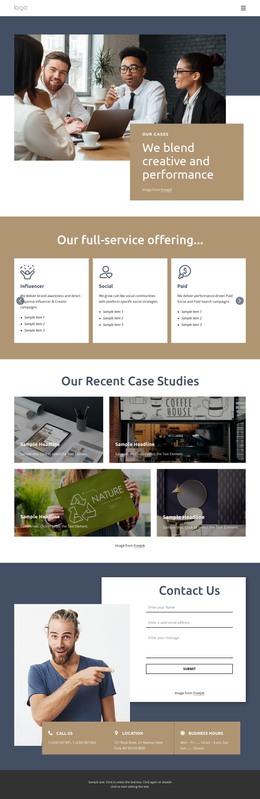This screenshot captures the vibrant and visually engaging website of a marketing, creative, and advertising agency. The image is vertically aligned, mimicking the experience of scrolling down through the website. Dominated by large, multicolored visuals featuring a palette of dark blue, beige, tan, green, white, and other hues, the site aims to be both eye-catching and informative.

At the top of the screenshot, there's an image showcasing a group of individuals in business casual attire seated around a table, likely discussing creative strategies or projects. This scene sets a collaborative and professional tone for the website. In the bottom right corner of the image overlay, a tan box with white text proclaims, "We blend creative and performance," summarizing the agency's mission.

Further down, a large tan box prominently displays in bold white text, "Our Full Service Offering." This section includes navigational links to various services provided by the agency, such as influencer marketing and social media management, among others.

Centering the middle of the screenshot, gray text introduces a segment called "Our Recent Case Studies." This area features four images, each depicting a project that highlights the agency's diverse capabilities. One image captures the lively atmosphere of a coffee house adorned with various coffee logos, while another showcases a person holding a green sign that reads "Nature" in white text, accompanied by a recycling logo—demonstrating the agency's involvement in environmentally conscious campaigns.

At the very bottom of the page, a dark blue box stands out with the text "Contact Us." This section provides fields for visitors to enter their phone number or email address to initiate further communication about the agency's services. Positioned to the left of this box is an image of a man in a blue shirt, pointing to the right towards the contact section, subtly guiding users to take action and reach out for more information.

The screenshot demonstrates the agency's emphasis on blending creativity with performance, offering comprehensive services while showcasing their past successes through visually rich case studies, and encouraging potential clients to contact them.